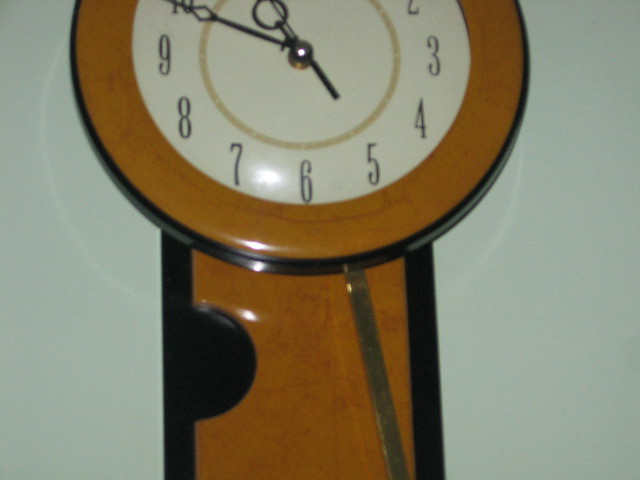This image features a real-life clock mounted on a wall painted in a very light sea green color. The clock is made of polished wood and is primarily circular in shape, though the top half is cut off in the image. This results in a view that includes only the lower half of the 2 and 10 numerals, but clearly displays the integers 3 through 9, which are written in serif font along the white background of the clock face.

The clock has a wooden border, and an additional smaller circle, outlined in a golden hue, is present on the inner part of the clock face. The clock's hands are elegant and metallic; the hour hand is a slim stick with a circular tip, while the minute hand is longer and ends in a diamond-like shape. Although the exact time is partially obscured due to the cut-off top portion of the clock, it can be roughly estimated to be around 11:50.

Beneath the clock face, there is a rectangular wooden slab that extends downward, featuring a black segment as part of its design. Affixed to this piece is a bronze pendulum that appears to be in mid-swing, adding to the clock's ornate appearance. However, the lower portion of the clock, including the end of the pendulum, is not visible in the image.